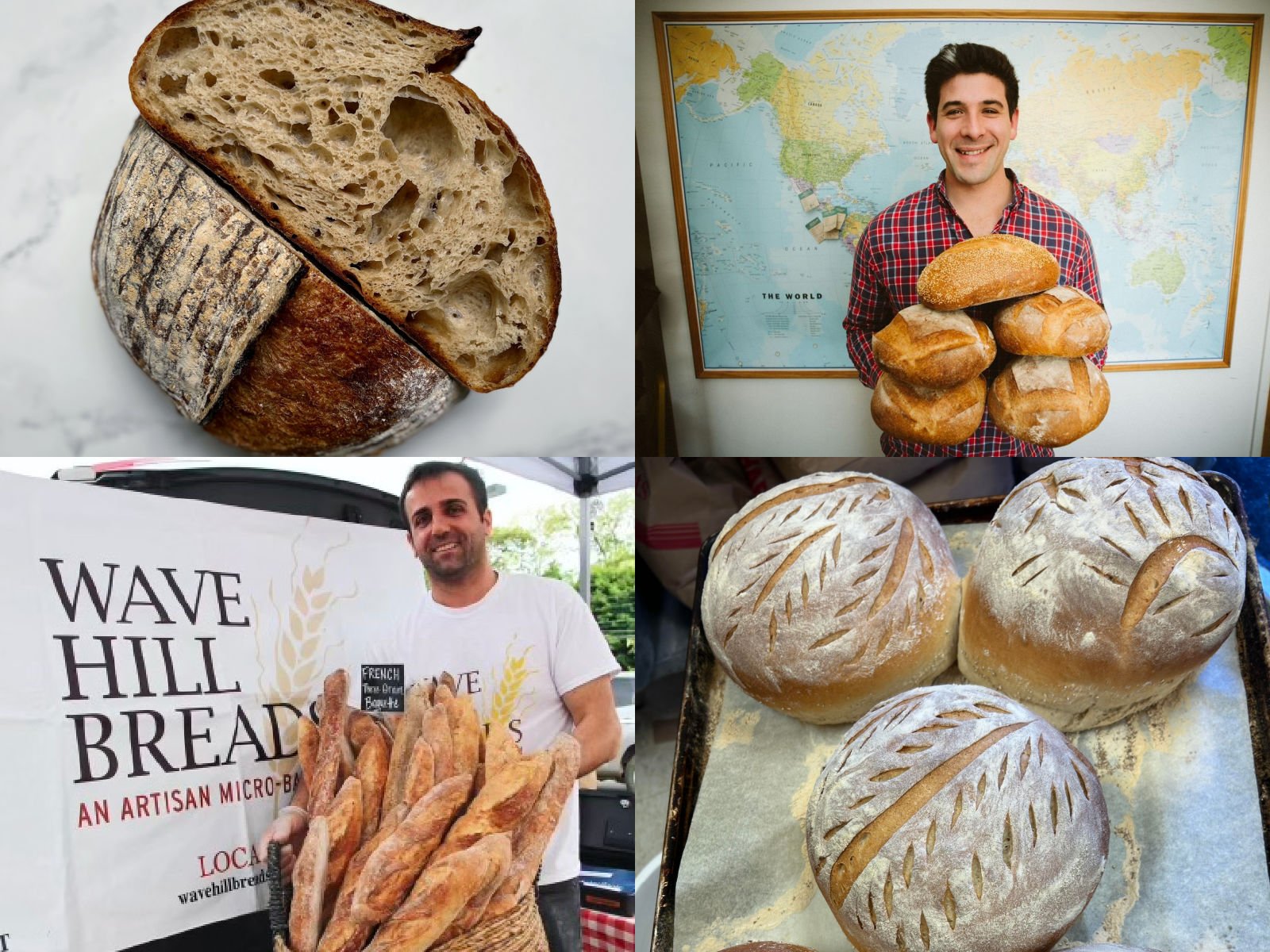The image is a collage divided into four sections, highlighting various aspects of Wave Hill Breads, an artisan micro bakery. In the top left quadrant, there is a close-up of a beige artisan loaf, sliced in half to reveal its interior, set against a gray, marble background. Beneath this, in the bottom left, is a cheerful man in a white t-shirt, emblazoned with the Wave Hill Breads logo, standing behind a basket brimming with large, flour-dusted artisan loaves. The t-shirt’s text is partially visible but matches the font of the bakery's sign, which reads "Wave Hill Breads, an artisan micro bakery, local," although the URL at the bottom of the sign is obscured. On the top right, another man, clad in a plaid shirt and standing in front of a map, holds five different loaves of bread. Finally, the bottom right section features an assortment of decorative bread loaves in a basket, capturing the rich browns and beiges of the freshly baked goods. The overall setting is photographic, with a detailed and warm depiction of the artisan craftsmanship of Wave Hill Breads. The color palette includes beige, brown, white, and hints of red, black, orange, green, yellow, and light blue, adding a vibrant touch to the artisanal theme.